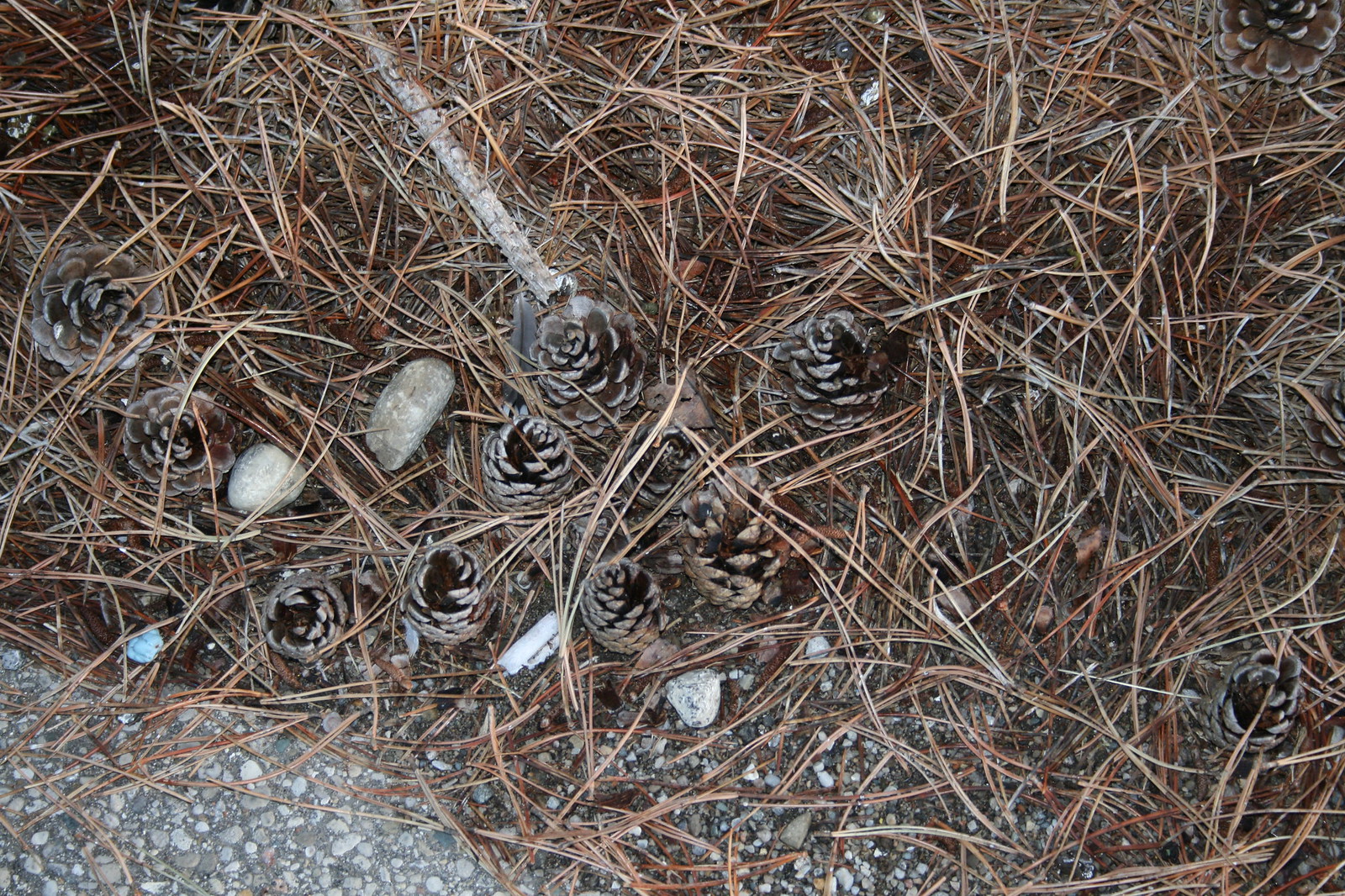The photograph is a close-up, top-down view of a ground surface scattered with various natural debris. Prominently featured are numerous medium-brown to dark-gray pine cones, which are mainly clustered in the center with a few scattered towards the edges. Many of these pine cones are standing on end, allowing a look down into their darker interior spaces where light is occluded. Interspersed among the pine cones are twigs and brown, dead pine needles, alongside reddish and brownish straw-like filaments. The ground is a mix of textures, with a noticeable difference in the lower left corner where a section of smoothed and darker gray material, possibly asphalt or some other composite substance, forms an angled edge. This smoother area contrasts with the surrounding pebbles, grit, and stones of various sizes, some of which are embedded into the ground while others remain loose. There is also a fragment of what appears to be a smashed cigarette butt among the debris, adding a touch of human impact to the natural scene.